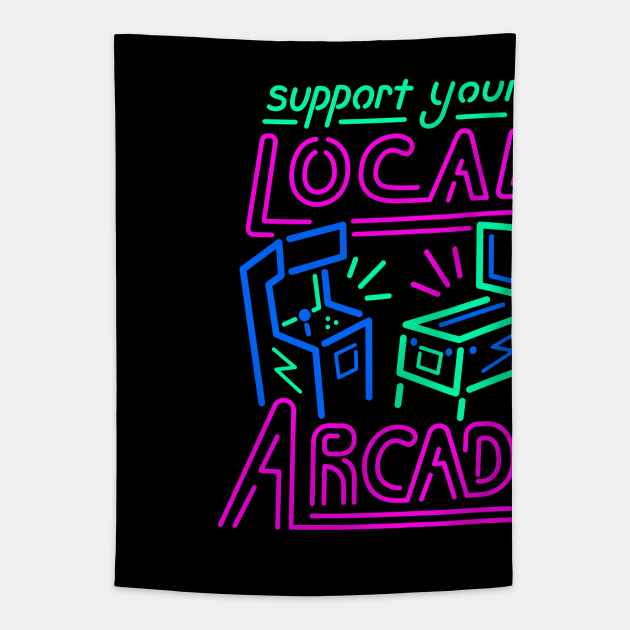The image, appearing as part of a poster or sign, is attached to a light gray wall and has a slight curvature around its edges, indicating it's loosely affixed. It features a vertical rectangular layout with a black background and is partially cut off at the right side and top. In a small, green neon font at the top, the text reads "support your," while a larger neon pink font spells "local," though the last letter 'L' is cut off. Below this, there are neon-colored illustrations of arcade machines; one appears to be an arcade cabinet with a joystick and buttons, and the other resembles a classic pinball machine. Beneath the illustrations, the word "arcade" is displayed in neon pink, missing the final 'E'. The illustrations of the games are outlined in green and blue neon, adding a vibrant touch to the encouraging message of supporting local arcades.